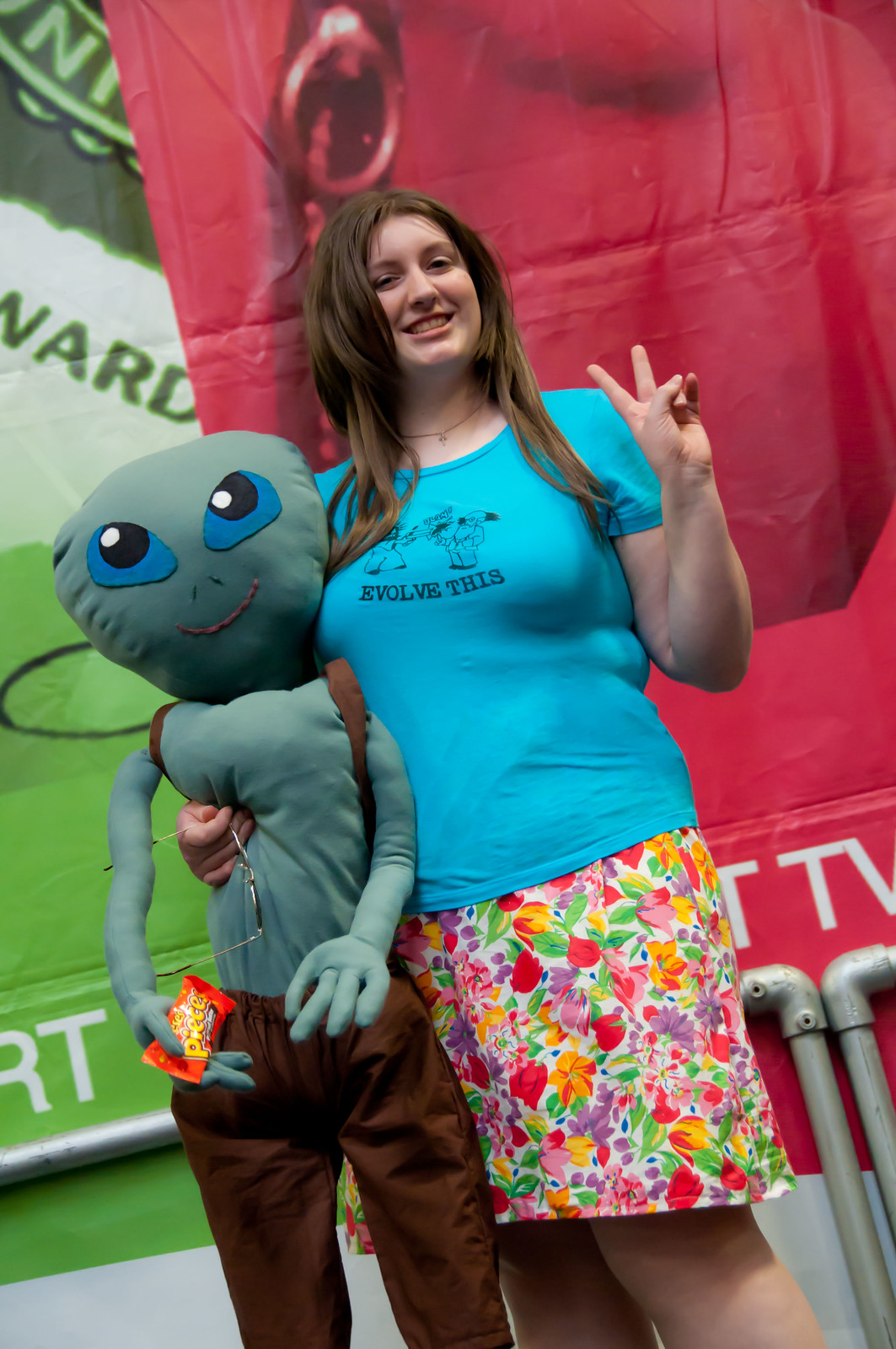In this vibrant and detailed image, a girl with long, reddish-brown hair that cascades down to her chest is smiling warmly at the camera. She is wearing a blue t-shirt with the phrase "Evolve This" emblazoned on it, paired with a floral skirt and white leggings. The girl is striking a peace symbol with her left hand and holding a smiling alien plushie with blue eyes and brown pants in her right. This plushie also has a brown backpack and clutches Reese’s Pieces in its right arm. She is positioned in the center of the photo, surrounded by an assortment of colors including gray, brown, red, pink, purple, green, yellow, orange, tan, light blue, various shades of green, white, and maroon. The backdrop features large banners, one red and one green, flanking either side of her, alongside some metal poles and gates. The scene appears to be set outdoors during the day, possibly at a convention, adding to the lively and engaging atmosphere of the image.